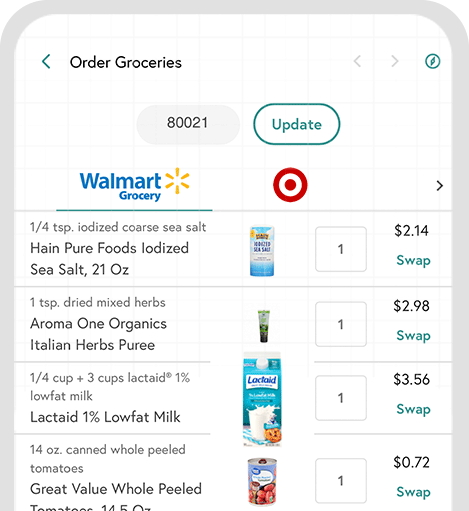A partial screenshot of a smartphone displaying a grocery ordering app interface. The visible portion of the phone has light gray borders framing the screen. Centered on the screen is an arrow pointing to the left with the label "Order Groceries". On the right side, there are two arrows—one pointing left and the other right—resembling a compass icon.

Below the arrows, there are two buttons: one labeled "80021" in a light gray highlight, indicating it's selected, the other labeled "Update" in white, indicating it's not selected. Underneath these buttons, the text "Walmart Grocery" appears next to the Walmart logo on the left and a circular icon resembling a target on the right.

Following this section, there are four product listings, each with an associated image and description. The first item is "Hand Pure Foods Iodized Sea Salt, 21 ounces," with a picture of the sea salt next to it. Details include a count of one and a price of $2.14, followed by an option to "Swap." This product listing format repeats with the subsequent items: "Aroma One Eggs," "Low Fat Milk," and "Great Value Whole Peeled Tomatoes."